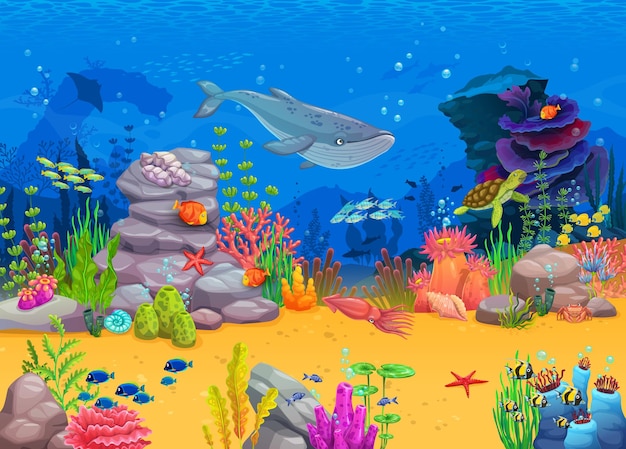This vibrant digital illustration features an enchanting underwater scene that could easily be from a children's book. The blue water is teeming with diverse sea life and colorful details. Dominating the center of the image is a majestic grayish-blue whale, flanked by a green sea turtle swimming ahead. Schools of fish in a variety of hues—light blue, orange, green, and some with black stripes—dart through the water. The ocean floor is a sandy expanse dotted with intricate rock formations, bright coral reefs in shades of blue, purple, red, and various other hues, along with clusters of seaweed and other underwater plants. Spotted among the flora are starfish, shrimp-like creatures, and a small pink squid. A shark can be seen chasing the turtle, while in the background, the faint shadow of a stingray adds depth to the scene. Bubbles scattered throughout the water add a playful touch, enhancing the illustration's appeal to young readers. The textures and colors are smooth and vibrant, contributing to the overall whimsical and children-friendly aesthetic.